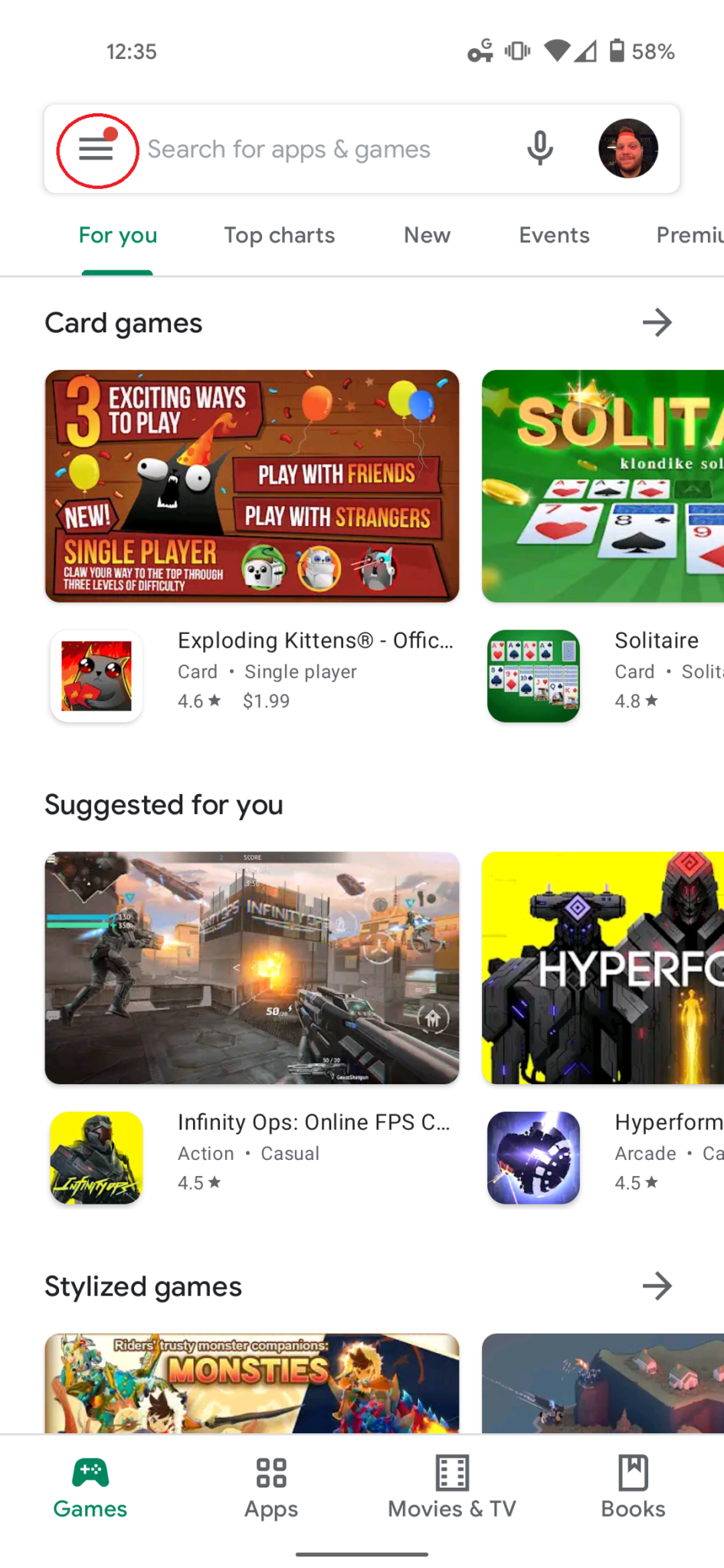The image appears to be a screenshot of a mobile application store interface. Here is a detailed description of the image provided:

**Top Bar:**
- *Top Left*: The time is displayed as "12:35."
- *Top Right*: There are several icons positioned sequentially:
  - A key-like icon with a circle over it.
  - A rectangle with lines extending from both sides.
  - A Wi-Fi symbol.
  - A triangle, darker on the left and outlined on the right.
  - A battery icon indicating 58% charge.
  
**Search and Navigation:**
- Below the top bar, a red circle surrounds three horizontal lines with a red dot on the top line.
- A search bar with the text "Search for apps and games" and a microphone icon.
- A circular icon with a person's face in it.
- A navigation tab underlined in green with the text "For You."

**Categories & Sections:**
- Navigation options next to "For You": "Top charts," "New," "Events," and a partially visible option that starts with "Preem."
- A horizontal gray separator line.

**Featured Apps & Games:**
- Section titled “Card Games” with an image showing the text: "Three exciting ways to play, new single player, play with friends, play with strangers," accompanied by balloons.
- Another image, partially cut off, likely titled "Solitaire," showing cards on a green background.
- An app icon for "Exploding Kittens®" which is partially readable: "O-F-F-I-C..." with additional details below.
- A description below the Solitaire icon.
- A "Suggested for you" section featuring:
  - An image depicting a war scene to the right, captioned "Hyper F..." with robots in the background.
  - A yellow square featuring a figure, labeled "Affinity Ops Online, F-P-S-C..." with further text below.
  - A purple square with a circular emblem, titled "Hyper Foam" with additional text.
  
**Stylized Games Section:**
- A partial image labeled "MONSTIES" with additional imagery.
- Another image featuring a building.

**Bottom Navigation:**
- Icons representing different categories:
  - A game controller icon for "Games" in green.
  - A four-square grid for "Apps."
  - A rectangle with dashes for "Movies & TV."
  - A rectangle with a bookmark for "Books."
- Another gray separator line at the bottom.

This comprehensive caption provides an in-depth description of the various elements of the interface, ensuring clarity and a detailed visual representation of the screenshot.